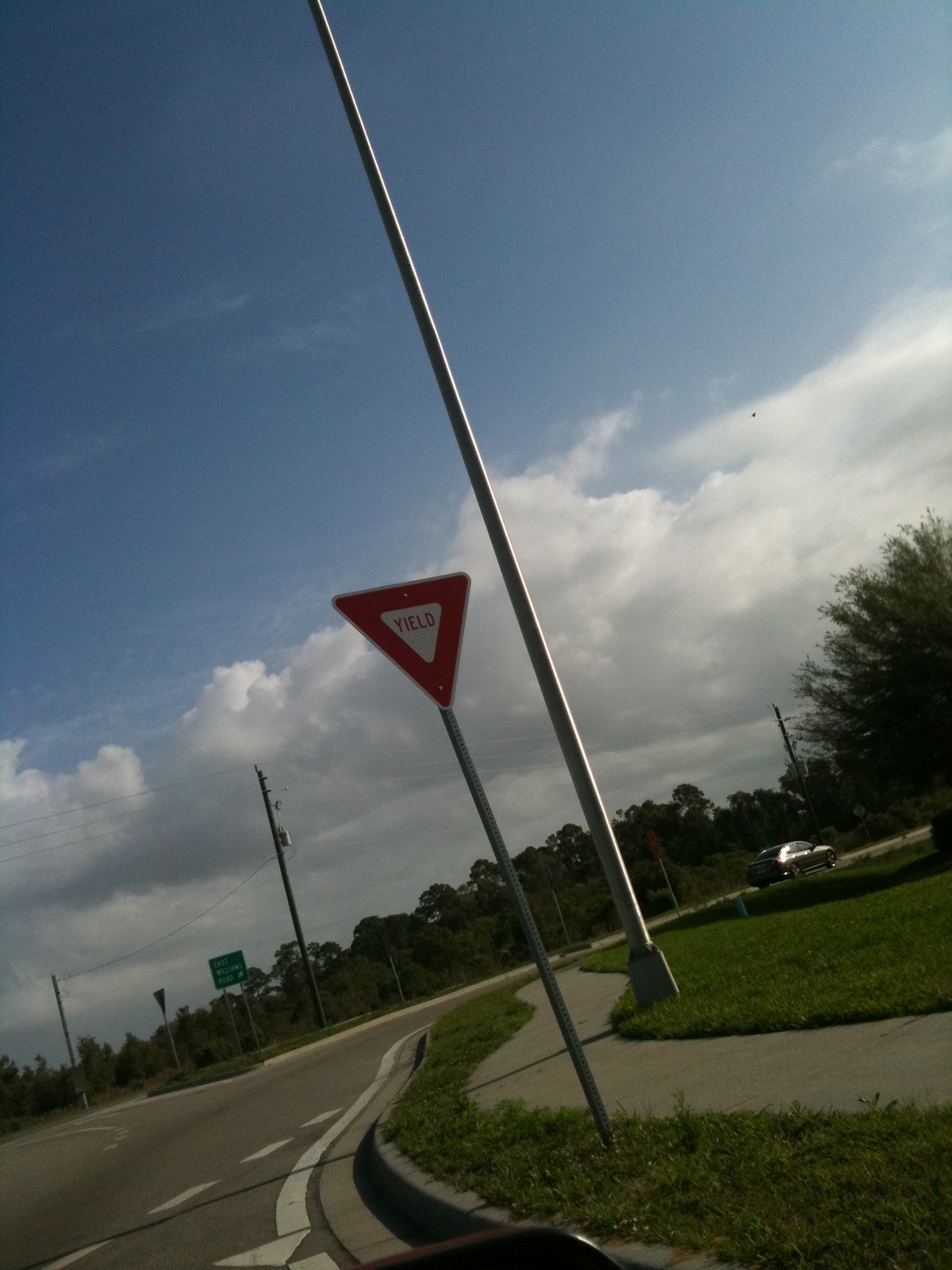The image captures a slightly tilted urban setting with a backdrop of clear, light-medium blue sky adorned with wispy clouds at the top and thick, fluffy cumulus clouds below. The lower half of the sky hints at potential rain with some darker patches in the distance. Below the cloud-filled sky, rows of trees with rounded, green tops line the background, adding a touch of nature to the scene. 

Prominent in the background is a green highway sign displaying information about the approaching city and its distance. To the left of this sign stands a yield sign, angled slightly to the left. Above, telephone lines stretch between three poles, marking their presence from the far left to the far right of the image.

In the midground, a car is captured driving to the right on a street or freeway, emphasizing the urban locale. In the foreground, there is a partial view of a pole, which is situated in the grassy area adjacent to a sidewalk. Beyond the sidewalk, another yield sign, characterized by its distinctive red and white triangular design and the word "YIELD" in red, stands on a gray pole embedded in the grass. This detailed arrangement of elements vividly portrays a scene where urban infrastructure meets the natural sky, all skewed slightly left due to the angled shot.